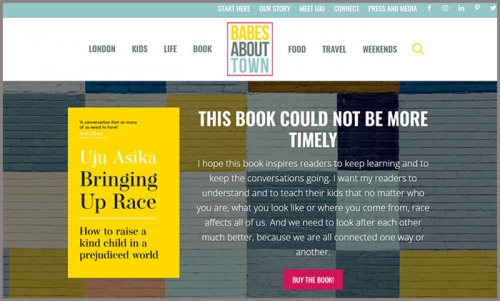**Detailed Caption:**

In the image, a website is displayed against a white background, featuring a light green header with a gray border. The header contains white text with tabs reading: "Start Here," "Our Story," "Meet," "Connect," and "Press and Media." Social media icons for Facebook and Twitter are also visible. Below the header, a central white banner showcases the main title, "Babes About Town," highlighted prominently.

Beneath this banner, navigation links are organized from left to right, reading: "London Kids Life Book," "Food," "Travel," and "Weekends," accompanied by a yellow magnifying glass icon. Further down, an image of a book with a yellow cover is presented. The book, titled "Raising Up Race: How to Raise a Kind Child in a Prejudice World" by Yuju Asika, stands out.

To the right of the book cover, white text provides a supportive review that reads: "This book could not be more timely. I hope this book inspires readers to keep learning and to keep the conversation going. I want my readers to understand and to teach their kids that no matter who you are, what you look like, or where you come from, race affects all of us, and we need to look after each other much better because we are all connected one way or another."